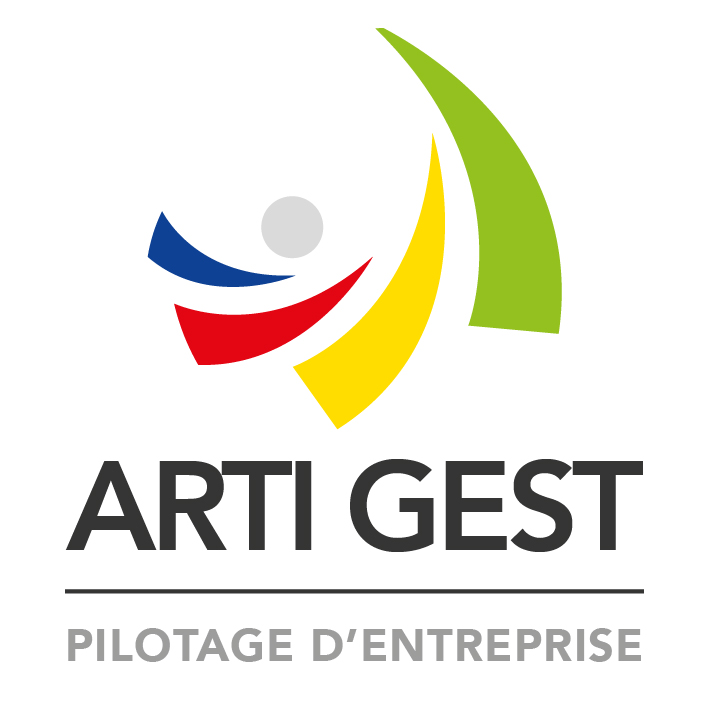The image displays a logo for a French company named "Artiguest." The top portion features a dynamic, circular design composed of four curved, pyramid-like shapes of increasing size, creating a sense of spinning motion. These shapes are distinctly colored in blue on the left, red below it, yellow to the right, and green above, all encircling a central gray dot. Below this vibrant motif, the text "Artiguest" is written in bold black font, separated by a horizontal black line from the subtext "Pilotage d'Enterprise" in smaller gray letters. The background of the logo is white, emphasizing the colorful and structured design.